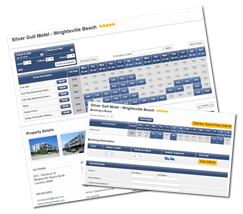A small screenshot of a calendar system, likely for the Silver Gulf Motel in Whiteville Beach with a five-star rating, dominates the image. The title at the top clearly reads "Silver Gulf Motel Whiteville Beach ★★★★★". Various small icons and options are meticulously arranged within the blue interface, including a blue options box and pictorial representations of parking lots and locations at the bottom. The main feature is a prominent blue bar stretching across the screenshot, annotated with months, indicating its function as a vacation planner. The background image appears skewed at an 8 to 10-degree angle to the right, while a second overlapping transparent box is similarly angled to the left. Together, they create a slightly disjointed visual but emphasize the detailed structure meant for planning monthly stays at the mentioned hotel.